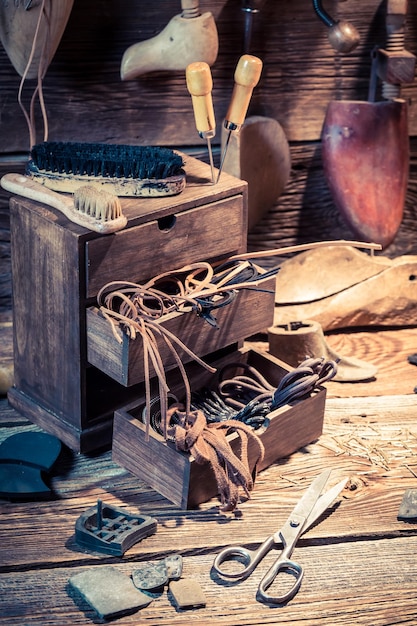The photograph showcases a meticulously cluttered workspace dedicated to leatherworking and shoe-making tools. Central to the image is a small, dark wooden chest of drawers, approximately a foot high and six inches deep. It sits on a wooden surface, under which lies a pair of large silver shears with metal handles. The middle drawer of the chest is open, spilling out numerous bundled leather cords and straps, while the bottom drawer, removed entirely, contains even more such materials. The top drawer remains closed. On top of the chest, there are two types of brushes: one with white bristles and a white handle, and another oblong brush with black bristles. Additionally, two metal pick tools are lodged on the top surface. The wooden wall behind the chest features various hanging tools, including what appear to be wooden shoe molds, essential for stretching and shaping shoes. The surrounding surface is strewn with an array of tools and smaller items related to leather crafting and shoe-making.